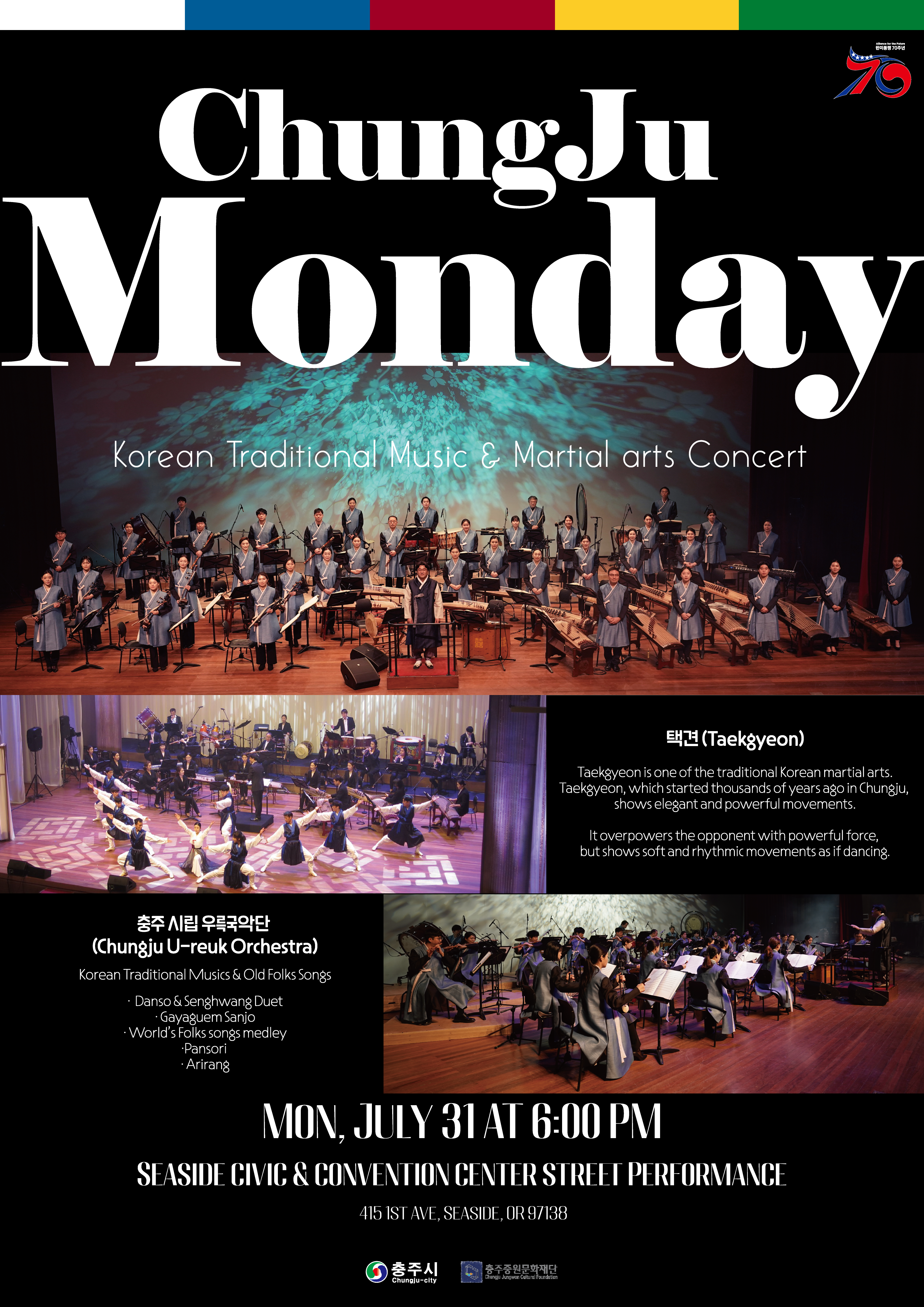This poster for the event titled "Cheongju Monday: Korean Traditional Music and Martial Arts Concert" is an advertisement that combines the visual elements of a color strip at the top and detailed text. The poster features a title in prominent white letters against a black background, along with a large image of a traditional Korean orchestra dressed in blue, black, and white uniforms, performing in front of a screen displaying soothing blue water visuals. The event showcases various elements including the Cheongju Ryeok Orchestra performing Korean traditional music, old folk songs, and specific numbers like a Danso and Sanghwang duet, Gayageum Sanjo, Pansori, and Arirang. Additionally, it highlights Taekyeon, a traditional Korean martial art known for its elegant yet powerful dance-like movements. The event takes place on Monday, July 31st, at 6 p.m. at the Seaside Civic and Convention Center, located at 415 First Avenue, Seaside, Oregon, zip code 97138.